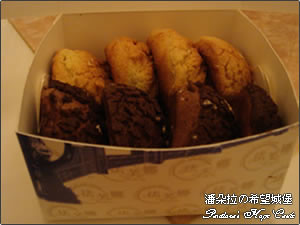The image depicts an open, reflective silver container with thin metallic sides. Inside the container, there are two rows of what appear to be pastries or baked goods. The top row contains four puff-style pastries that are light golden brown, while the bottom row has four chocolate pastries with sprinklings on them. These pastries are arranged upright on their sides, possibly resembling biscuits or cookies. The container, likely made of cardboard, features a circular pattern around its interior. At the bottom of the image, there is some small, blurred text with Chinese characters and some pixelated English lettering that is difficult to read.